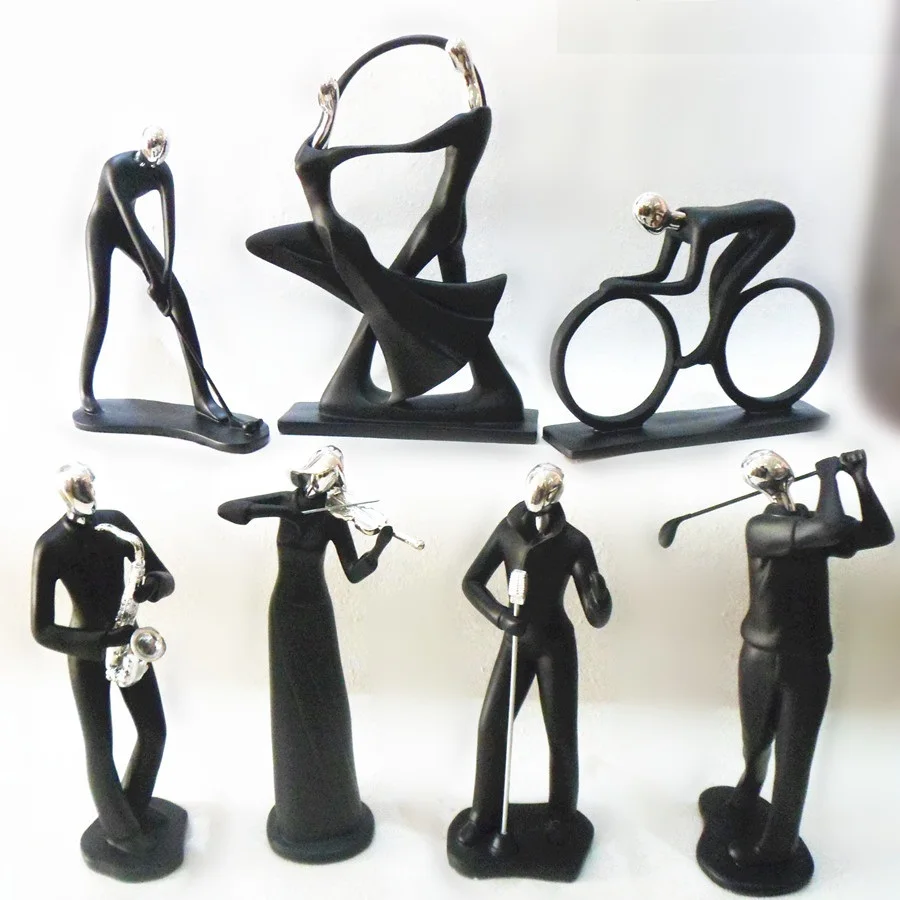The image features a collection of seven black and silver figurines, each meticulously designed to represent individuals engaged in various activities. All the figurines, which differ slightly in body type—from thin to muscular to heavier set—are posed dynamically against a stark white background. The figurines are organized in two rows; the top row contains a man bent over, about to tee off with a golf club, followed by a dancing couple with elongated necks, and then a man on a bicycle with no axle or spokes. The bottom row starts with a man playing a silver saxophone, a woman in a long evening gown playing a silver violin, a figure holding a retro square silver microphone, and finally, a heavier set man completing a powerful overhead golf swing. Each figure's head is silver, and they cast subtle shadows, adding depth to the otherwise monochromatic scene. The image lacks any text and showcases minimal color variations, emphasizing the contrast between the white background and the black-and-silver figurines.